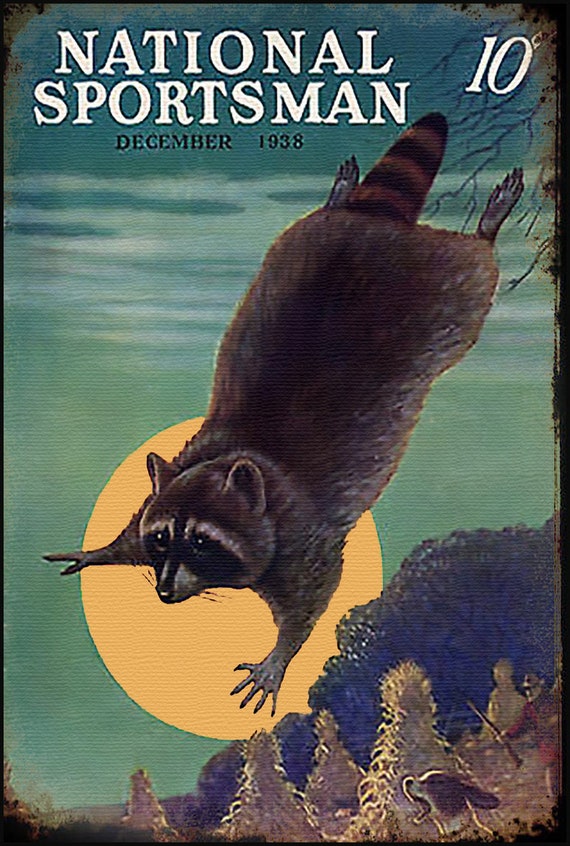This image, possibly a cover for a magazine, book, or even a stamp, prominently features the bolded title "National Sportsman" in white text at the top left corner, with "December 1938" just below it. The price, "Ten Cents," is marked in the top right corner. The central illustration vividly portrays a chubby raccoon leaping off a tree, with its arms outstretched and its ringed tail visible. Behind the raccoon, either a moon or a setting sun illuminates the sky, which is a mix of beige and blue hues, interspersed with white clouds. The background reveals a dense forest scene, with additional details including what appears to be a beagle or similar dog with an open mouth, positioned at the bottom right. This dog is possibly barking at the raccoon. Nearby, possibly behind the dog, there is a human figure holding a gun, suggesting a hunting scene. Sparse tree branches extend into the frame from the top right, adding depth to the rustic outdoor setting.